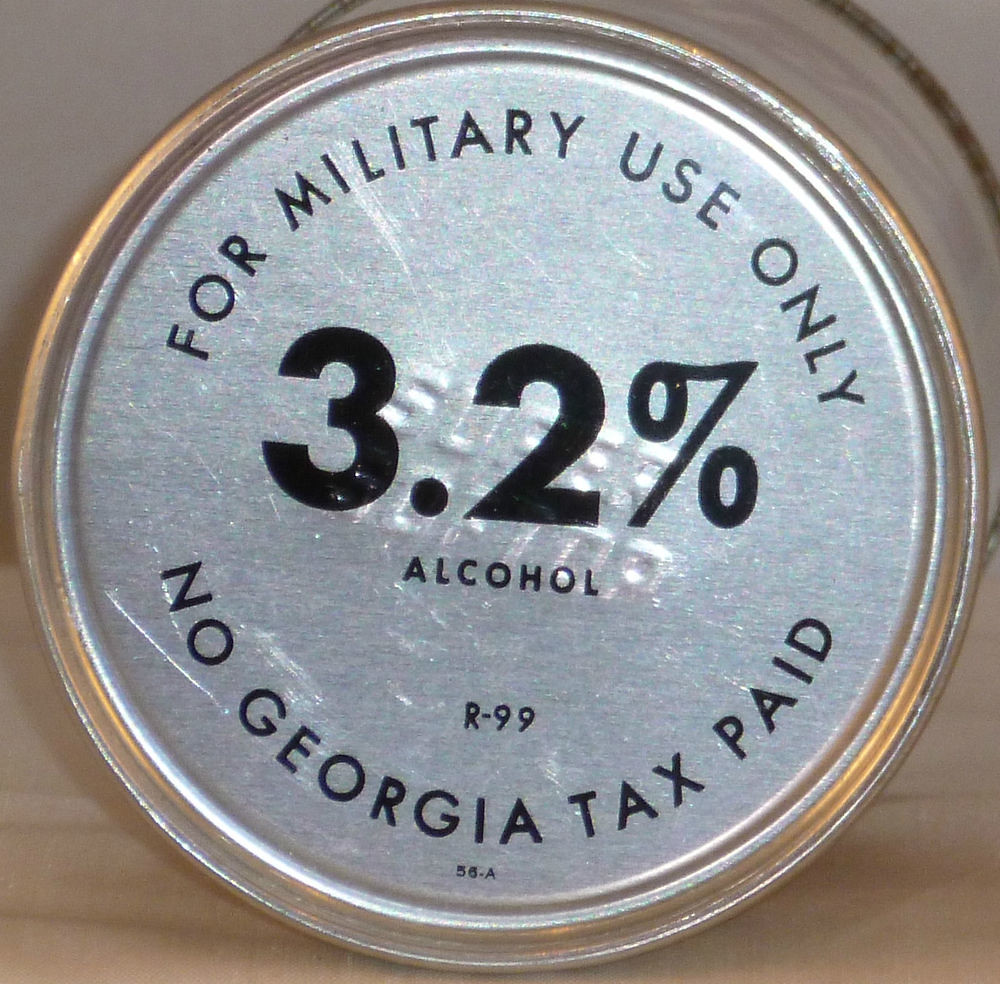The photograph depicts a silver aluminum can lying on its side on a light blonde wood table. The visible bottom of the can is inscribed with black lettering. At the top of the arc, it reads "for military use only," while the continuation of the text states "no Georgia tax paid." In the center of the bottom, the marking "3.2% alcohol" is prominently displayed, accompanied by the notation "R-99" which might be a code. This indicates the can likely contains a beverage, possibly an army-issued beer due to its low alcohol content, and is tax-exempt due to its military use designation.